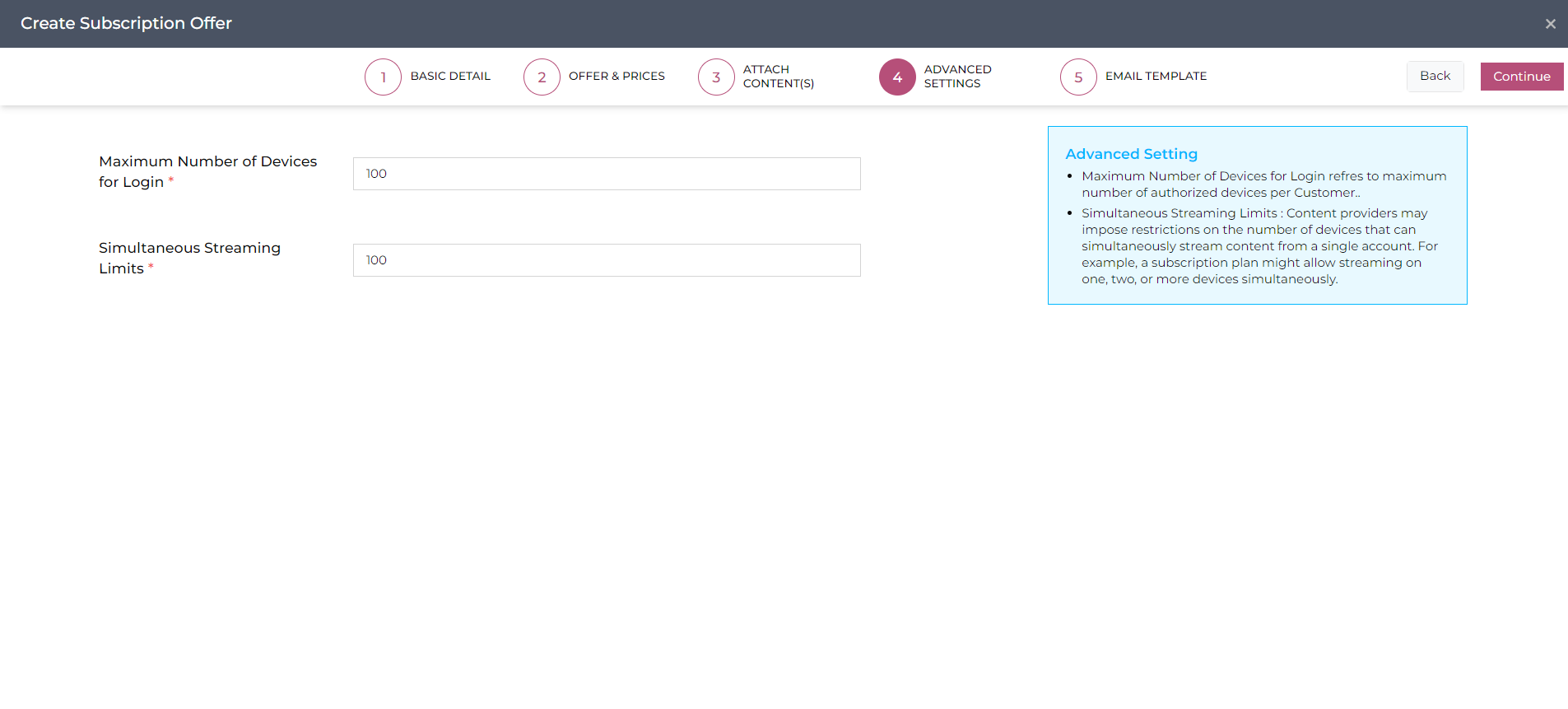**Caption:**

The webpage section displays the Advanced Settings for a subscription offer. The top part features a dark grey banner with the title "Create Subscription Offer" in white text, and an "X" at the far right corner to close the window. Below this banner, five numbered and labeled circles track the progress of the setup process: 1) Basic Detail, 2) Offer and Prices, 3) Attach Contents, 4) Advanced Settings, and 5) Email Template. The fourth circle, representing the Advanced Settings, is highlighted in magenta.

On the right side, there are two buttons: "Back" and "Continue." The "Continue" button is also highlighted in magenta.

Directly beneath the banner on the left side, two settings boxes can be seen: "Maximum Number of Devices for Login" and "Simultaneous Streaming Limits," both set to 100. Towards the right, a light blue enclosed box titled "Advanced Setting" has two bullet points explaining the settings: 1) "Maximum Number of Devices for Login" refers to the maximum number of authorized devices per customer, and 2) "Simultaneous Streaming Limits." The "Continue" button appears here in a magenta box.

The overall space below the banner is white, and there are no borders on the sides or bottom.